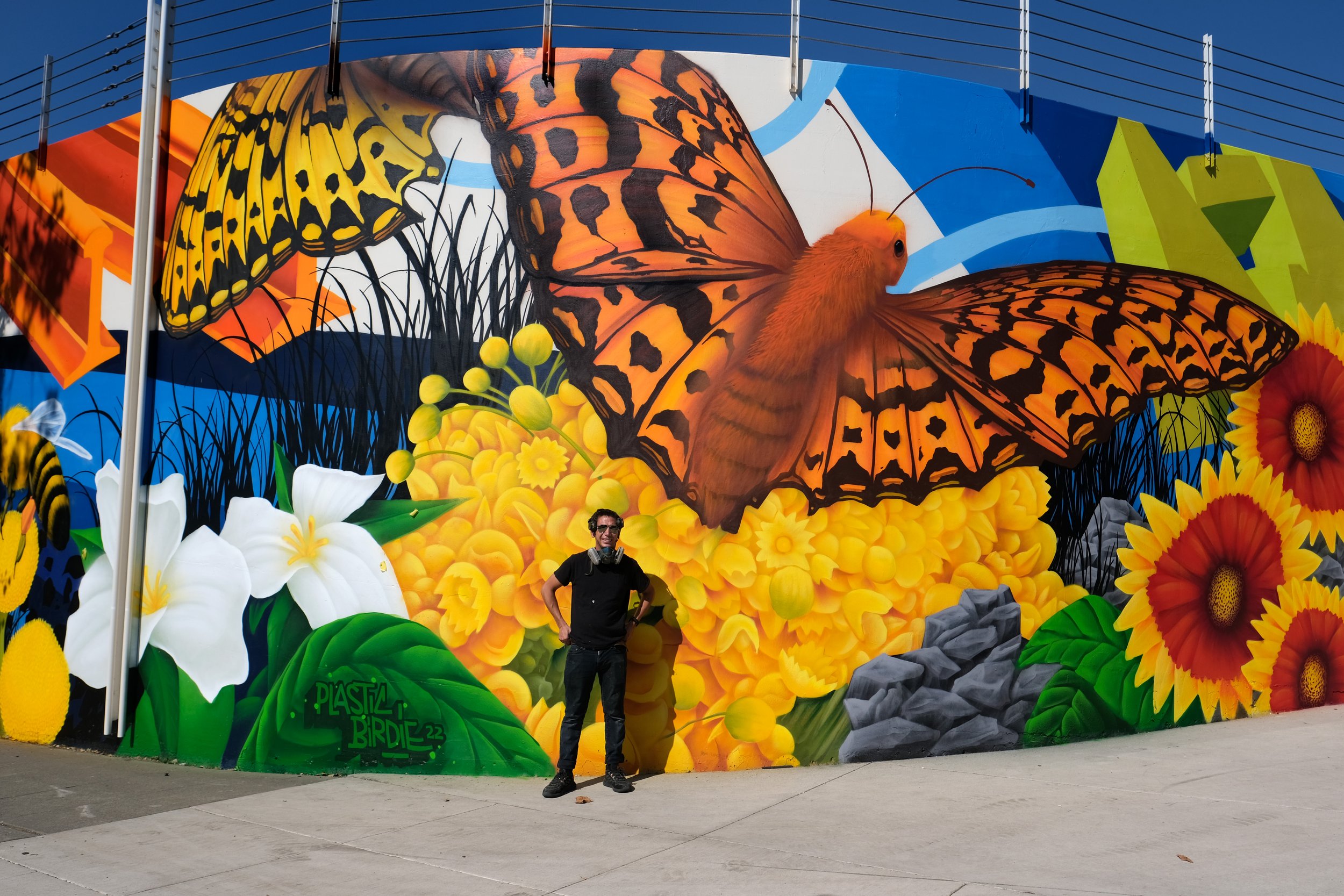The image captures a vibrant outdoor scene featuring a man standing on a light gray concrete sidewalk in front of a massive, colorful mural on a concrete barrier. The mural, possibly extending up to 18 feet high, is intricately detailed and spans the background, showcasing an artistic blend of nature and urban elements. The man, dressed in a dark short-sleeve polo shirt, dark pants, and black shoes, stands confidently with his hands on his hips, suggesting he may be the artist. 

The mural is a vivid tapestry of colors and themes. Dominating the left side are blooming white flowers with yellow centers, while to the right, a strikingly large orange butterfly appears to be in flight, moving upwards and to the right. Surrounding this butterfly is a field of small yellow flowers. Above, a yellow butterfly's left wing is visible, flying over two depicted orange I-beam girders. Adjacent to these elements are three large sunflowers with green leaves, and a patch of small rocks illustrated nearby. Embedded within the lush, green leaf on the mural is the inscription "Plastic Birdie 22."

Further back, the mural features a greenish-yellow architectural design against a backdrop that transitions through shades of blue and white, possibly representing the sky with hints of urban structures. The entire piece exudes a sense of harmony between nature and urban life, all captured with sharp, realistic detail in the photograph.